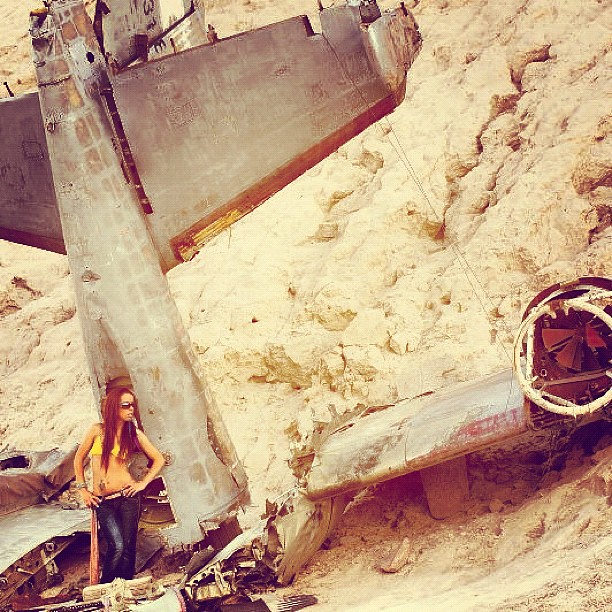The color photograph captures a dramatic scene that appears to be either a work of art or a stylized modeling photo. Central to the image is the crashed remains of an airplane, with its nose buried in the sandy hillside, its tail and part of the wings jutting out at awkward angles. The aircraft is grey and bears the number "31" towards its aft section. The surroundings include a steep, brown rocky cliff that ascends sharply behind the plane.

Standing near the fuselage is a slender, young adult woman striking a confident pose. She is wearing a yellow bikini top paired with low-rise black hip-hugger pants, showcasing her midriff and secured with a silver or white belt. Her dark, reddish-brown hair falls freely across her chest. She accessorizes her look with large, dark sunglasses and holds a bat with her left hand, leaning on it casually. The woman stands with one hip slightly out, hands placed on her hips, and gazes to her left. The scene is brightly lit, indicative of natural daylight, adding to the stark contrast between the vibrant human figure and the wrecked, desolate airplane.